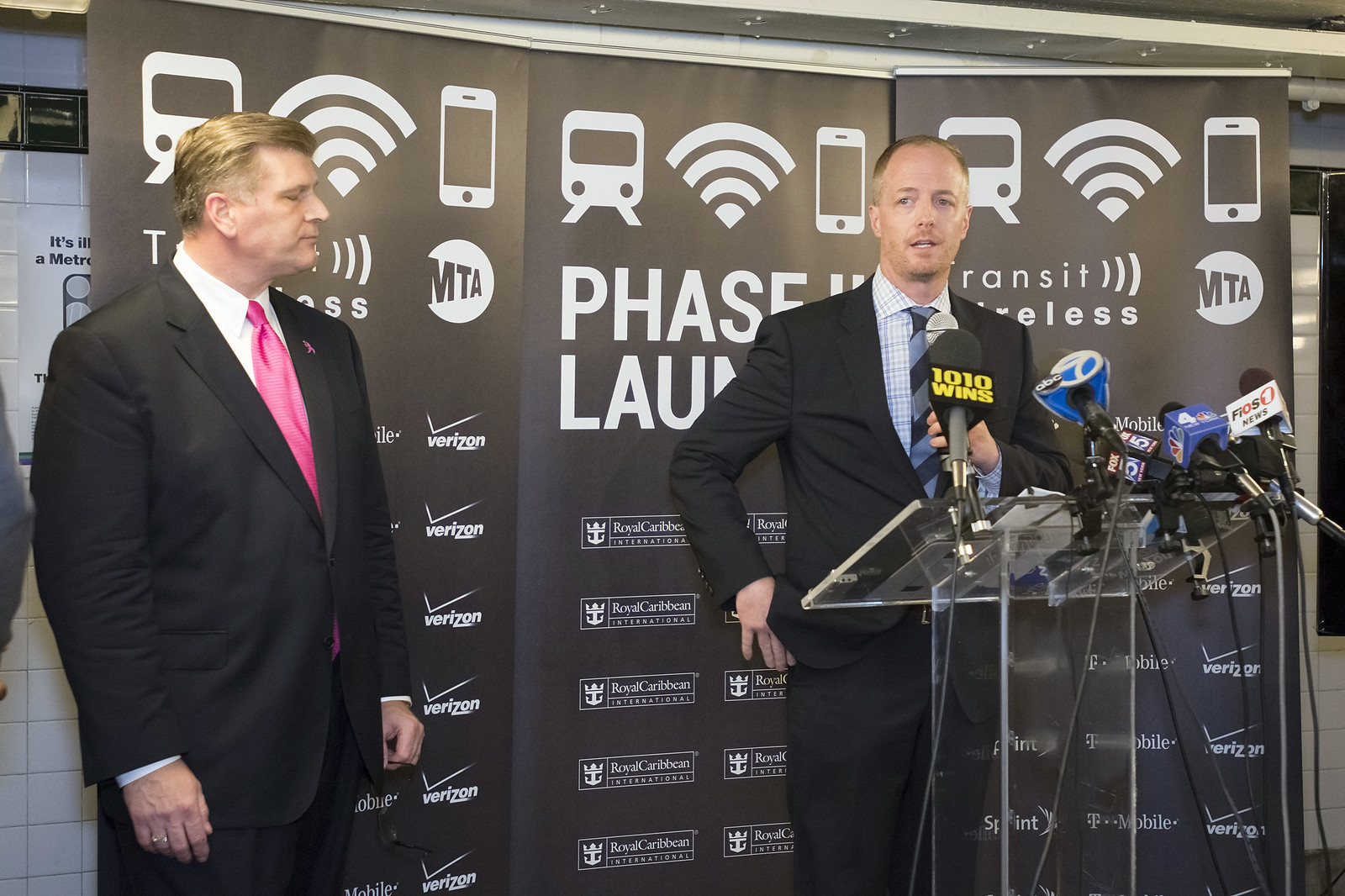In the photograph, two men stand in front of a banner emblazoned with logos from various organizations such as Verizon, Royal Caribbean, MTA, and Sprint. The central figure, positioned slightly to the right, is a Caucasian man with very short brown hair, dressed in a black suit, black pants, a blue and white plaid button-up shirt, and a dark blue and black striped tie. He is at a clear, tilted podium bristling with an array of microphones from major networks including ABC, Fox, NBC, and local affiliates. His hand appears to be on or near a microphone labeled with "1010 WINS" in gold lettering. The second man, further to the left, has slicked-back blonde hair and seems to have his eyes closed while looking slightly toward the center. He wears a black suit, black pants, a white collared shirt, and a pink tie. The backdrop features various images such as a subway cart, a WiFi logo, and a phone silhouette amidst the corporate logos.